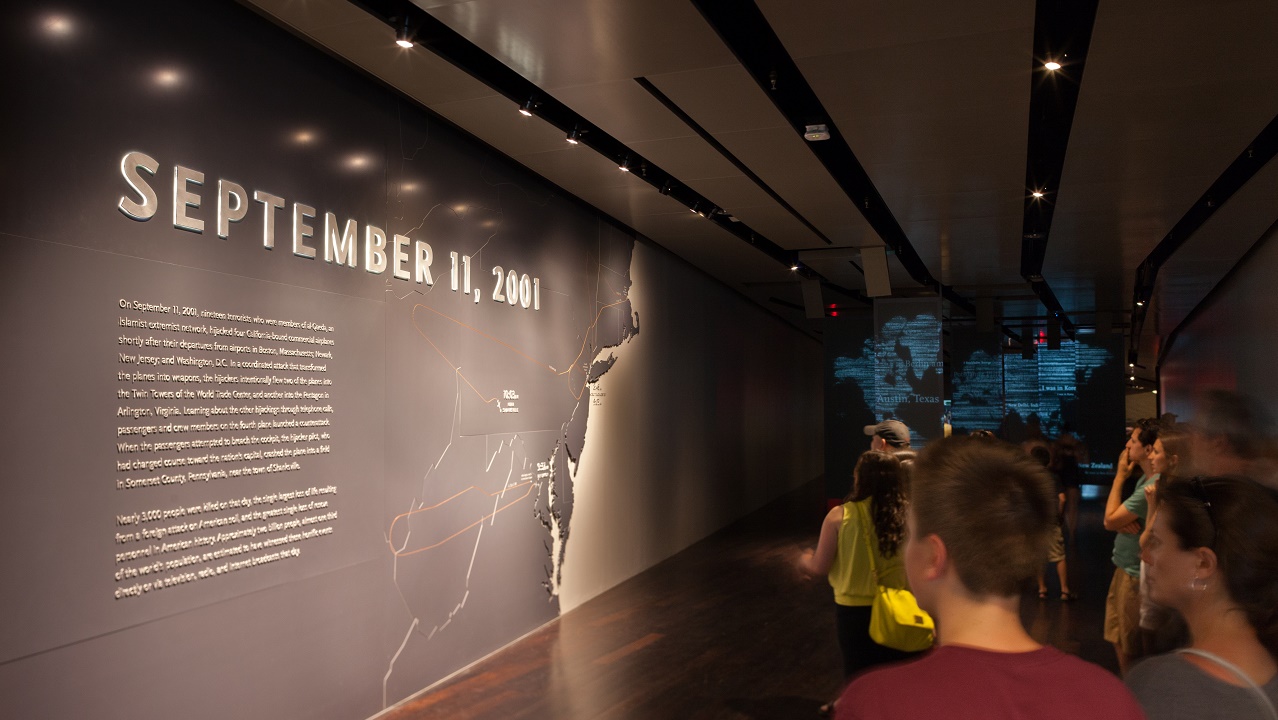The photograph captures a solemn exhibit at a museum dedicated to the events of September 11, 2001. Dominating the scene is a large mural occupying a significant portion of the wall, depicting the eastern coast of the United States in individual grayish tiles for each state. Below the prominent inscription "September 11, 2001," smaller, unreadable text outlines historical context, accompanied by a map detailing the flight paths of the hijacked planes. The museum's interior is dimly lit, with small, rounded ceiling lights casting a subdued glow over the exhibit. On the far wall, another display featuring illuminated blue maps and globes can be seen. Observers—comprising families and individuals, including a man with his hand to his mouth and a woman who appears to be emotional—gaze intently at the mural. In the foreground, the back of a student wearing a maroon shirt is visible, enhancing the educational and reflective atmosphere of the exhibit.